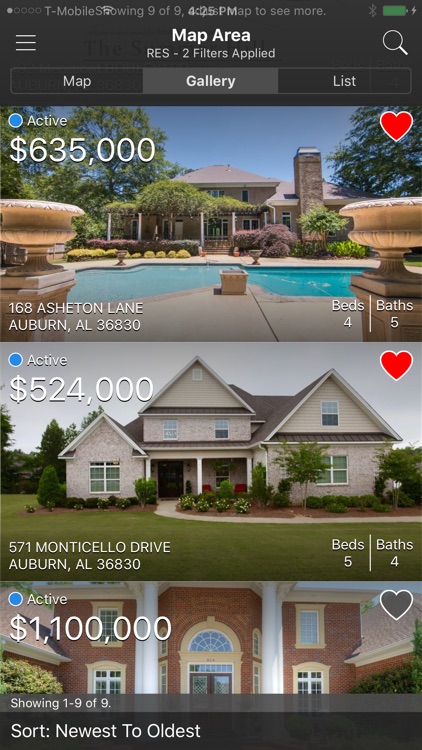The image showcases a user interface for a real estate application with several key sections and details. At the top, there's a text overlay reading "Map Arena Rest - Two filters applied," written in white against a black background. Below this header, three tabs are visible: "Map" on the left, "Gallery" in the center, and "List" on the right. The "Gallery" tab is highlighted in grey, indicating it is currently selected.

Beneath the tabs, the gallery view displays three property listings. 

1. The first listing features a house at 168 Ashton Lane, Auburn, AL 368, priced at $75,000. The house is marked as active by a blue dot on its left. The property has four bedrooms and five bathrooms. The image shows a light-colored house with a swimming pool in front, surrounded by trees. A red heart icon on the right signifies the listing is favorited.

2. The second listing is for a house at 57 Monticello Drive, Auburn, AL 368, priced at $24,000. Also marked as active with a blue dot, this property has five bedrooms and four bathrooms. The image depicts a house with slightly elevated walls, black roofing, green plants, and a concrete driveway. A red heart indicates this house is also favorited.

3. The third listing is for a property priced at $1,100,000. This house is also marked as active with a blue dot. The heart icon on the right is grey, indicating it is not favorited. Text below this listing indicates it is showing "one of nine" with a sort order from newest to oldest.

The distinct elements such as pool details, house descriptions, price points, and icons (blue dots, hearts) offer a clear and comprehensive overview of the selected properties.